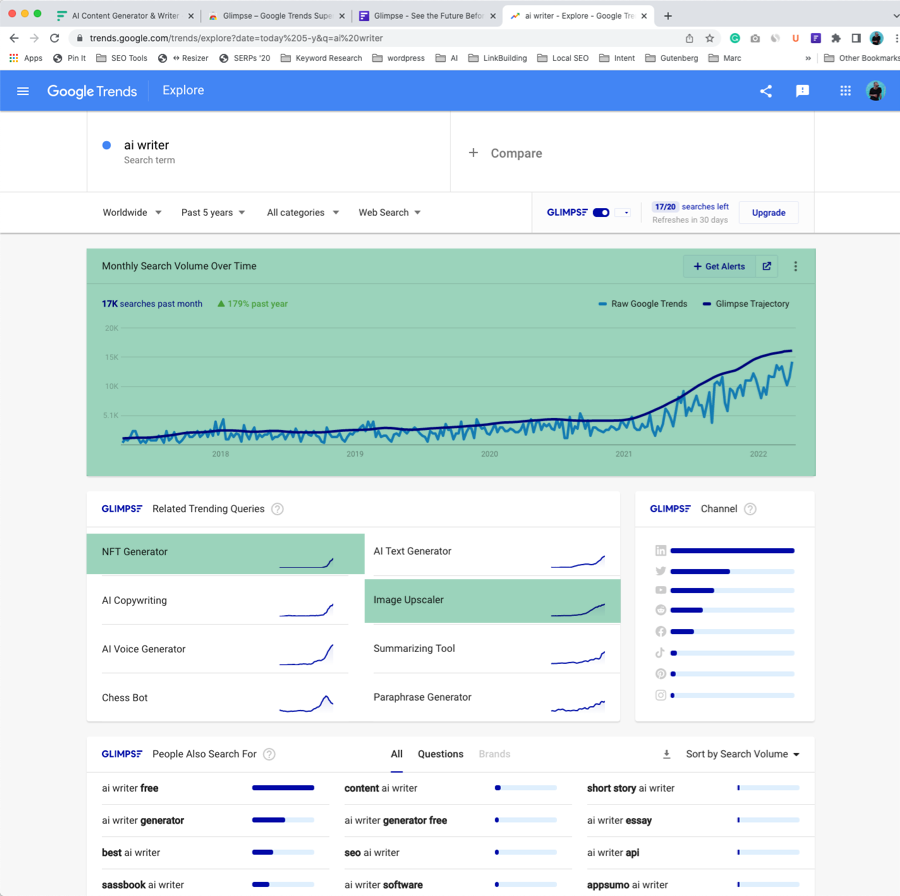This image is a detailed screenshot displaying various elements of a browser window filled with tools and information related to SEO and AI content generation. At the very top of the screenshot, multiple browser tabs are visible, including "AI Content Generator," "Glimpse," another "Glimpse" tab, "AI Writer," and "Explore Google." 

Directly beneath the tabs, the address bar shows the URL "Trends.Google.com." Below the address bar, a row of bookmarks stretches across the screen from left to right, featuring icons and names such as "Apps," "Pin It," "SEO Resizer," "SERPs20," "Keyword Research," "WordPress," "AI," "Link Building," "Local SEO," "Intent," "Gutenberg," and "Mark," among others.

A blue banner labeled "Google Trends" spans the width of the screen, with an "Explore" button and a small circular photo of a man wearing a black t-shirt and sunglasses located on the right side. Below this banner, a section dedicated to "AI Writer" displays a graph depicting monthly search volume over time. Beneath the graph, there is a section for "Glimpse" which lists various related trending queries.